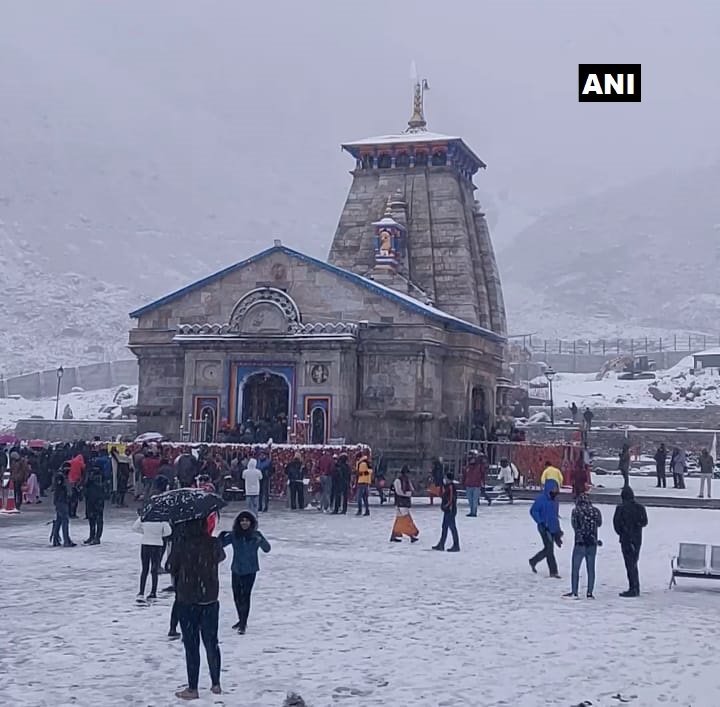In this vertically rectangular, full-color photograph, we see a serene winter wonderland setting captured during the daytime under overcast skies. A thick fog blankets a mountainous background, rendering the peaks barely visible. The ground is carpeted in a pristine layer of snow, adding to the ethereal atmosphere. People, dressed warmly in jackets, gloves, and scarves, with some even holding umbrellas to shield themselves from the falling snow, populate the lower part of the image. They appear to be casually walking around or engaged in quiet conversations, not part of any official activity.

The central focus of the image is a large, ornate brick church adorned with vivid colors—orange, blue, red, and yellow—particularly noticeable on its windows, main entrance, and a monument atop the roof. A red fence immediately surrounds the church, with numerous people visible both inside and outside its perimeter. Additionally, a black rectangle with white text reading "ANI" (also interpreted as "Annie" in the top right corner) adds a subtle digital touch to the image. Overall, the photograph beautifully captures a tranquil moment in a fog-covered, snowy landscape, highlighting the church as a beacon of color and community amidst the winter scene.